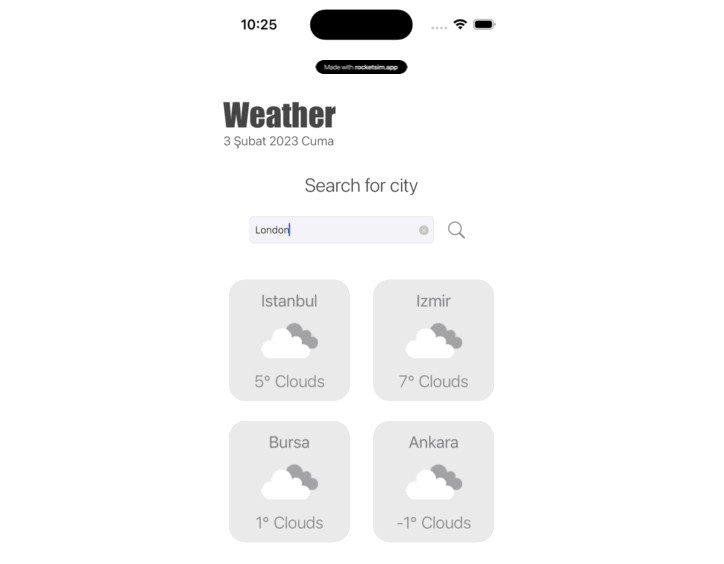The image shows a smartphone screen captured in portrait format. At the top left corner, the time "10:25" is displayed. Adjacent to the right are the Wi-Fi symbol and a black battery icon. Below these icons, written in a white text over a black oval shape, is the phrase "Made with RocketSim.app".

In large grey letters below, the word "Weather" is prominently displayed. Following this, "3 Subat 2023" and "Cuma" (which means "February 3, 2023 - Friday" in Turkish) are written in grey. Underneath this date information, there is a grey search bar with the text "Search for city" where inside, in darker grey text, the word "London" is pre-entered along with a blue blinking cursor.

To the right of the search bar, a magnifying glass icon is present indicating the search function. Below this, there are four sections, each displaying weather information for different cities with respective icons and labels. 

1. **Istanbul**: Shows a grey cloud with a white cloud overlay and the text "5° Clouds".
2. **Izmir**: Depicts the same cloud icon with "7° Clouds".
3. **Bursa**: Displays the cloud icons with "1° Clouds".
4. **Ankara**: Shows the cloud icons with "−1° Clouds".

Each city is represented with consistent iconography indicating cloudy weather and varying temperatures.